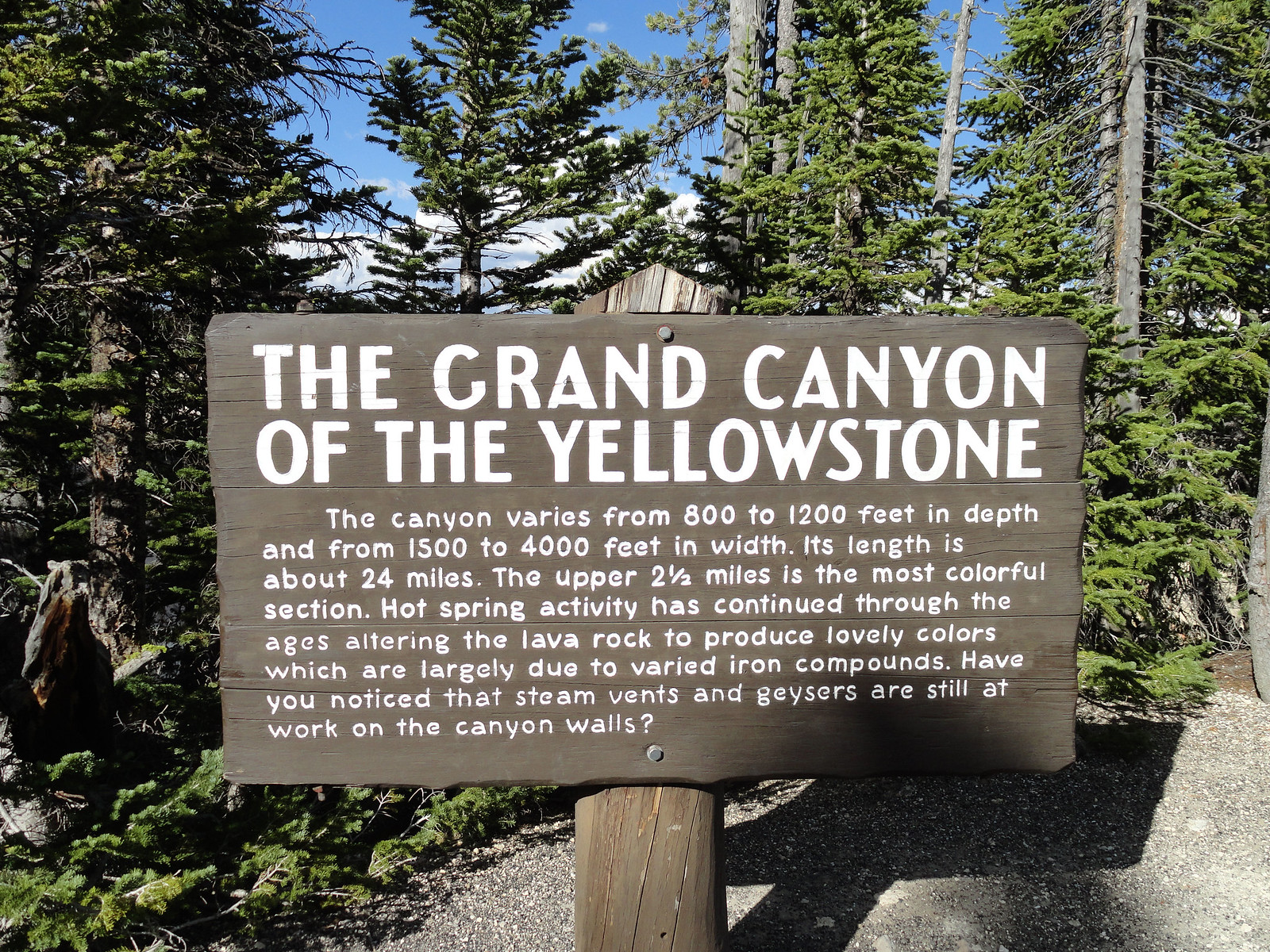On a partly cloudy day, this photograph captures a gray wooden sign with white text, prominently reading in all caps "THE GRAND CANYON OF THE YELLOWSTONE." Nailed to a sturdy brown wooden post by two silver nails, the sign provides detailed information about the canyon: "The canyon varies from 800 to 1200 feet in depth and from 1500 to 4000 feet in width. Its length is about 24 miles. The upper 2.5 miles is the most colorful section. Hot spring activity has continued through the ages altering the lava rock to produce lovely colors which are largely due to varied iron compounds. Have you noticed that steam vents and geysers are still at work on the canyon walls?" Behind the sign, a tranquil scene unfolds with a myriad of green trees with brown and white trunks and branches, set against a light blue sky adorned with fluffy white clouds. The ground in the foreground is a gravel-strewn area, and you can see bushes and grass sprouting vibrantly. Sunlight bathes the sign, casting a shadow behind it, enhancing the texture and detail of the surrounding natural setting.